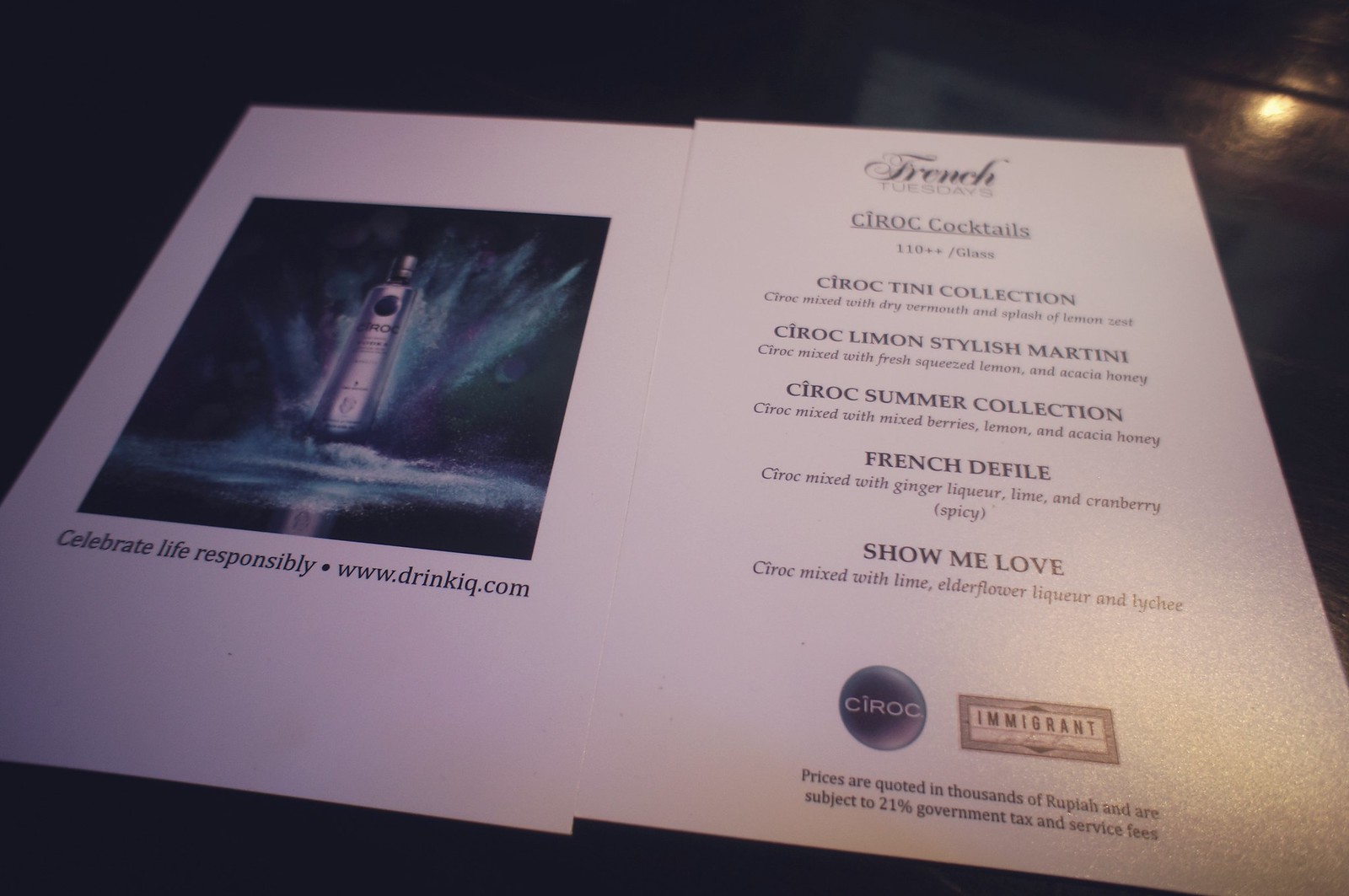The photograph captures a cocktail menu displayed on a dark, shiny surface. The menu is spread across two pages: the left page prominently features an image of a Ciroc vodka bottle, set against a black background with dynamic splashes of blue and purple water. Below this artistic visual, a white border at the bottom of the page bears the tagline "Celebrate Life Responsibly" along with the website www.drinkiq.com in black text.

On the right page, the cocktail menu itself begins with the heading "French Tuesdays." 'French' is written in cursive black font, with 'Tuesdays' in smaller black font below it. The menu lists a variety of Ciroc cocktails, including "Ciroc," the "Ciroctini Collection," "Ciroc Limon Stylish Martini," "Ciroc Summer Collection," "French Defile," and "Show Me Love." Each cocktail entry includes detailed ingredients, all in black text. Toward the bottom of this page, there is the Ciroc logo—a dark circle with "Ciroc" written in white within it. Additional text notes that prices are quoted in thousands of rubles and are subject to a 21% government tax and service fee, all in small black font.

Overall, the white background of the pages contrasts with the dark surface, emphasizing the clean and stylish presentation of the menu items.